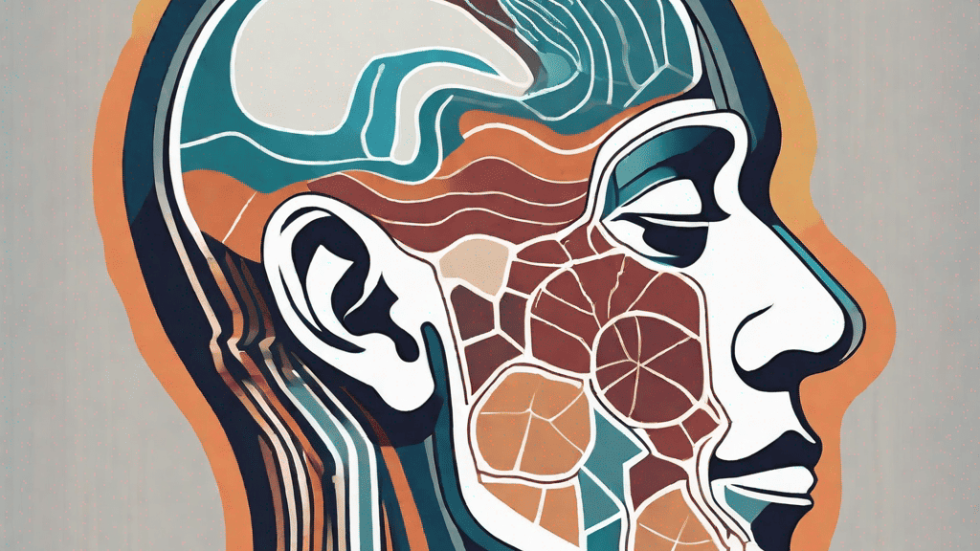This detailed and colorful cross-sectional illustration of a human head, shown from the side, reveals various anatomical features and layers through distinct colors and patterns. The image highlights the right side of the face, adorned with an orange halo outlining the entire head. The nose and eyelids are depicted in white, while the bottom lip is also white, contrasting with the black top lip. The eye appears closed and carries a marble-like texture with vibrant colors around the cheek area.

The brain region is predominantly shaded in blues, oranges, and reds, and is positioned above a tan and dark brown area. Various colored lines—orange, brown, teal, and white—cascade vertically down the back of the neck, indicating muscle structures. The ear, outlined in black, retains a flesh color. The cheek muscles are marked in red and orange hues, emphasizing their location right behind the eyes, contributing to the overall dynamic and vibrant composition.